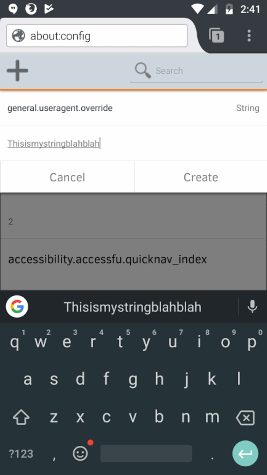The image appears to be a vertical screenshot from a web browser on a mobile phone, showcasing a detailed view of its interface. At the very top of the screen, familiar system icons are visible against a dark gray banner. On the right side, the Wi-Fi icon, cellular signal icon, a half-filled battery icon with a lightning symbol indicating charging, and the current time displayed as 2:41 can be seen. On the left side, there are several app icons, including a chat bubble, the Firefox browser icon, and an icon resembling a play button with a check mark in the middle, possibly from the Play Store.

Below this banner is the web browser interface. The address bar reads "about:config," indicating the configuration settings of the Firefox browser are being accessed. Next to the address bar is an icon indicating there is one open tab, represented by a single number "1" on overlapping squares, followed by a menu icon composed of three vertical dots.

The main content of the page is framed within a light gray banner holding a plus sign on the top left and a search bar with a magnifying glass icon on the right. Just below this, a thin yellow line separates the banner from the rest of the content. 

A heading labeled "journal.useragent.override" is displayed prominently, with the word "string" positioned to its right. Beneath this heading, is a user input field where the text "thisismystringblahblah" is being typed in a continuous, underlined format without any spaces. Accompanying this field are two action buttons: a 'Cancel' button on the left and a 'Create' button on the right.

Further down, a grayed-out section contains the number "2" followed by the text "accessibility.accessfu.quicknav_index.” The on-screen keyboard is visible at the bottom of the screenshot, indicating active text input.

This meticulously detailed caption offers a comprehensive view of the mobile browser's settings interface and the ongoing interaction.